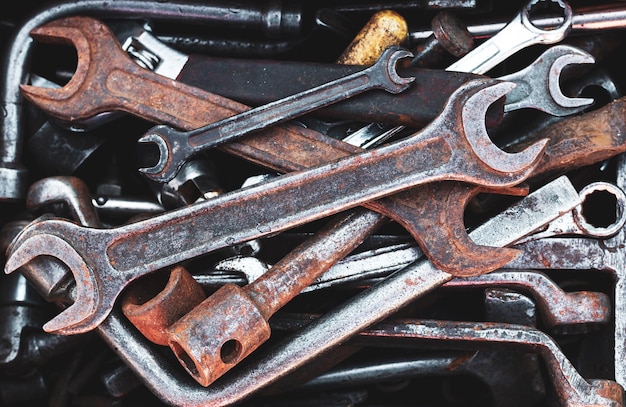The image depicts the interior of a vintage, heavily used, and soiled black toolbox filled with an assortment of tools. Dominating the pile are various wrenches, including both open-end and closed-end types, all of which show significant signs of rust and extensive use. Among them, a crescent wrench with an insulated handle, marred from wear, stands out. Peeking from beneath the array of wrenches, you can also identify the handle of a socket wrench and what appears to be a hammer. Additionally, extensions for socket wrenches and a possible crowbar, though partly obscured, are visible. The tools vary in size and functionality, and the overall scene is clearly captured in natural light, enhancing the visibility of the rust and grime that tell the story of their extensive use over time. There are no people or text in the image, just a vivid, close-up view of the tools meticulously laid atop one another.